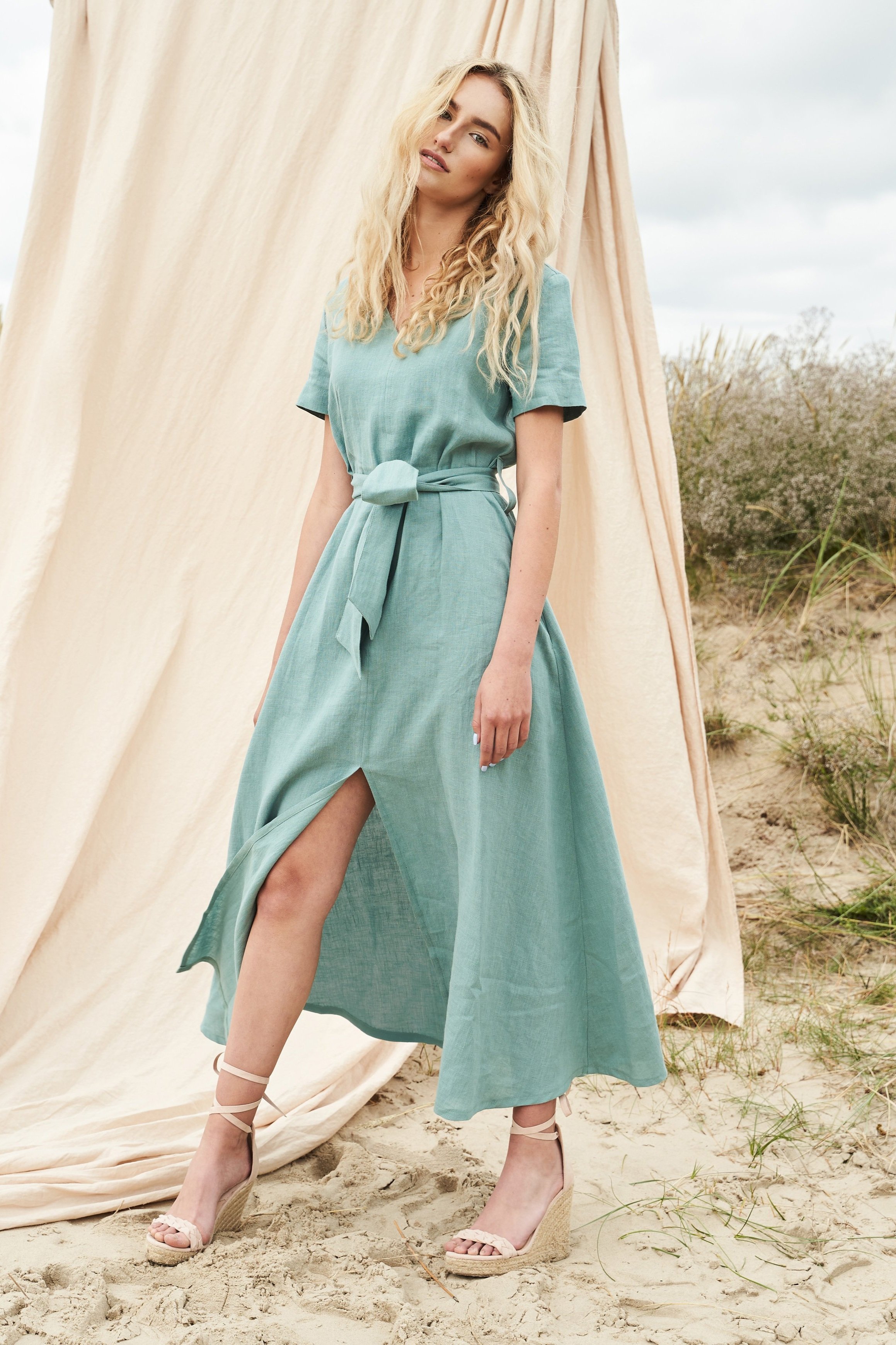In this vertically aligned rectangular color photograph, a model stands poised in a sandy beach area adorned with scattered blades of grass and small bushes. Dominating the background to the right is a stretch of tall weeds or bushes beneath a cloudy, gray-white sky that extends into the upper right and upper left corners. The model is positioned in front of a hanging beige drape or curtain, though the support for the drape is out of the frame.

The model, a blonde woman with long, curly hair cascading past her shoulders, tilts her head gently towards her left shoulder while gazing toward the camera. Her expression is neutral, with slightly parted lips. She is dressed in a striking, pretty green dress that falls to her ankles, featuring a cinched waist with a tied sash and a front slit that reveals her legs up to mid-thigh. Complementing her attire, she wears high-heeled sandals that have ivory straps wrapping around her ankles and tan wedge heels. Her fingers showcase white nail polish, adding a touch of subtle elegance to her overall look.